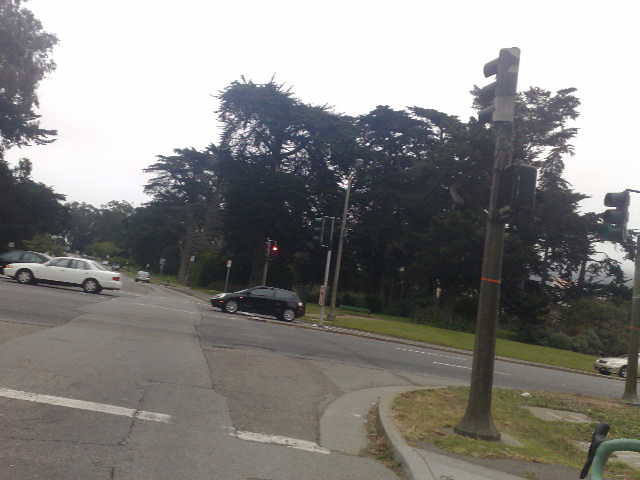The image is a color photograph of a somewhat busy city intersection on a cloudy, hazy day. The perspective is from a car standing at a red traffic light on the right side near the curb—just before the corner of the road. The scene is slightly wider than it is tall by about 20%. In the foreground, the crosswalk stretches horizontally, though its white painted lines are partially worn off, revealing the gray concrete beneath.

There are multiple black traffic light poles with red lights visible, one prominently placed in the lower right corner, oriented toward the 11 o'clock position. The intersection shows a white sedan, likely an older Toyota Camry, followed by a small black sedan, both positioned to turn left. Another white car is observed about 40% up the image, also heading left. The intersecting road extends straight and then curves to the left, suggesting at least two lanes allowing the left turn, but a right turn is either suggested or restricted.

The background features numerous tall trees with dark green leaves, adding to the urban yet slightly natural scenery. Additional street signs and possibly a bench are faintly noticeable, underscoring the pedestrian-friendly environment without visible pedestrians. The overall atmosphere illustrates an urban street scene captured in the middle of the day.